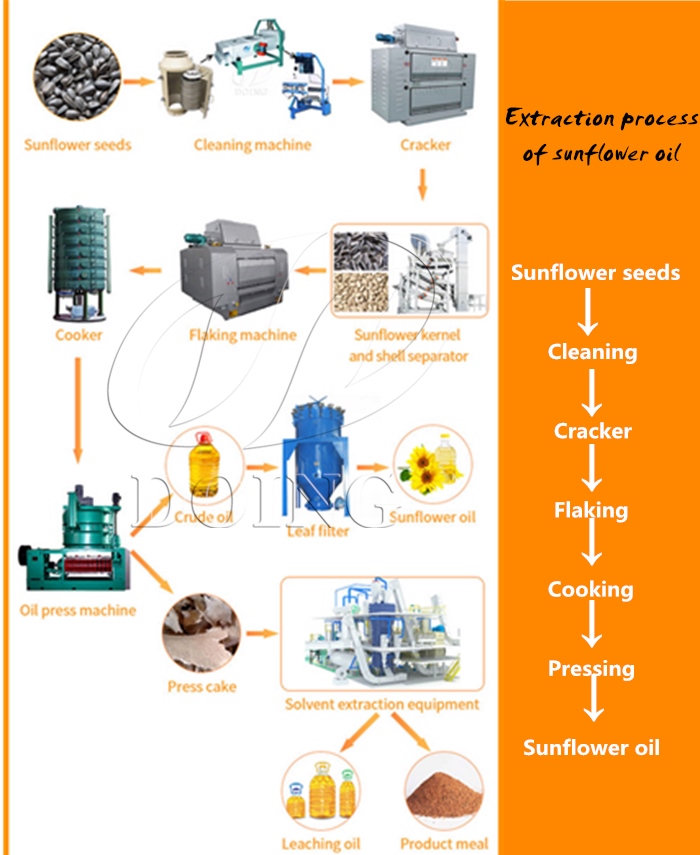This document features a detailed poster or flyer illustrating the extraction process of sunflower oil. The right-hand side of the poster showcases an orange-yellow vertical strip with black text outlining each step of the process: "Extraction Process of Sunflower Oil." Below this header, an ordered list follows: "Sunflower Seeds," "Cleaning," "Cracker," "Flaking," "Cooking," "Pressing," and finally, "Sunflower Oil," with each step connected by downward-pointing arrows.

On the left-hand side, the poster places various small illustrations corresponding to each step of the process described on the right. Starting from the top, it includes:

1. **Sunflower Seeds**: A drawing of black sunflower seeds.
2. **Cleaning Machine**: Depictions of three nondescript machines.
3. **Cracker**: A gray machine resembling a copier.
4. **Sunflower Kernel and Shell Separator**: An illustration indicating the separation process.
5. **Flaking Machine**: A drawing of a large piece of machinery.
6. **Cooker**: A cylindrical green apparatus.
7. **Oil Press Machine**: A greenish-blue machine responsible for extracting the oil.

Lastly, the outcomes of pressing are detailed with images: a bottle of crude oil and a by-product labeled "Press Cake." The crude oil image flows to a "Leaf Filter" and then to the final product, "Sunflower Oil," symbolized by a sunflower graphic. There's also a segment on "Solvent Extraction Equipment," highlighting a large machine, which leads to two additional drawings labeled "Leaching Oil" (depicted with bottles of oil) and "Product Meal" (shown as brown powder). This comprehensive visual guide intricately maps out how sunflower seeds are transformed into sunflower oil, emphasizing both the processes and the machinery involved.